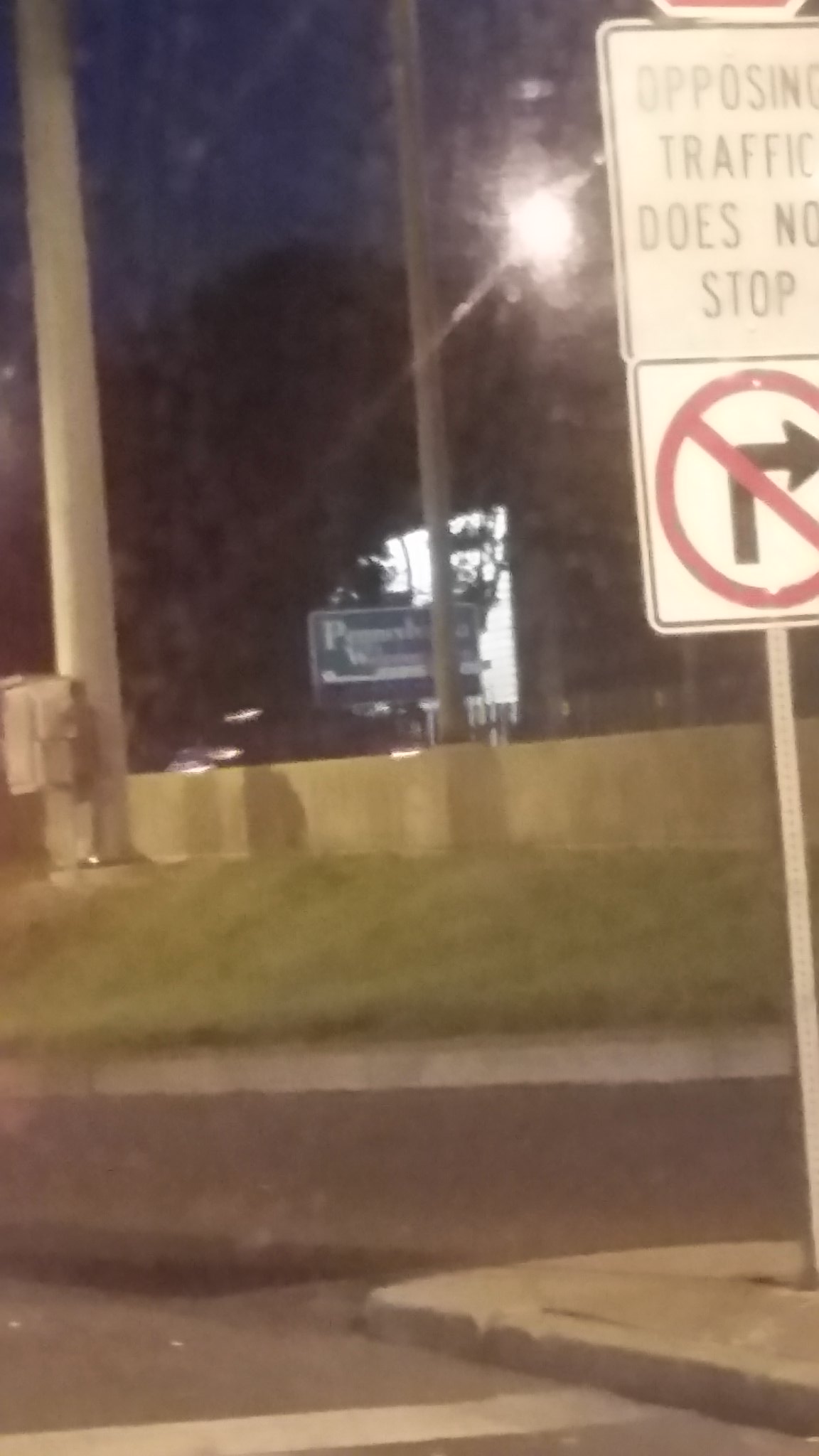This somewhat blurry, nighttime color photograph depicts an intersection taken from the road, showcasing various elements that detail the scene's layout. On the right-hand side, there is a concrete sidewalk island with a pole featuring two traffic signs. The upper white sign states "opposing traffic does not stop," while the lower sign has a right-turn arrow crossed out by a red circle with a diagonal line, indicating that a right turn is prohibited. The asphalt road, marked with a horizontal white line, extends into the distance, bordered on the left by a concrete barrier. Further back, amidst the dark sky and the silhouette of trees, a street light shines, and a large green sign is visible. The scene includes a black pole directly in front, possibly for street lighting, accompanied by another tall concrete light pole. The dim lighting and shadows emphasize the nighttime ambiance, obscuring finer details in the background.